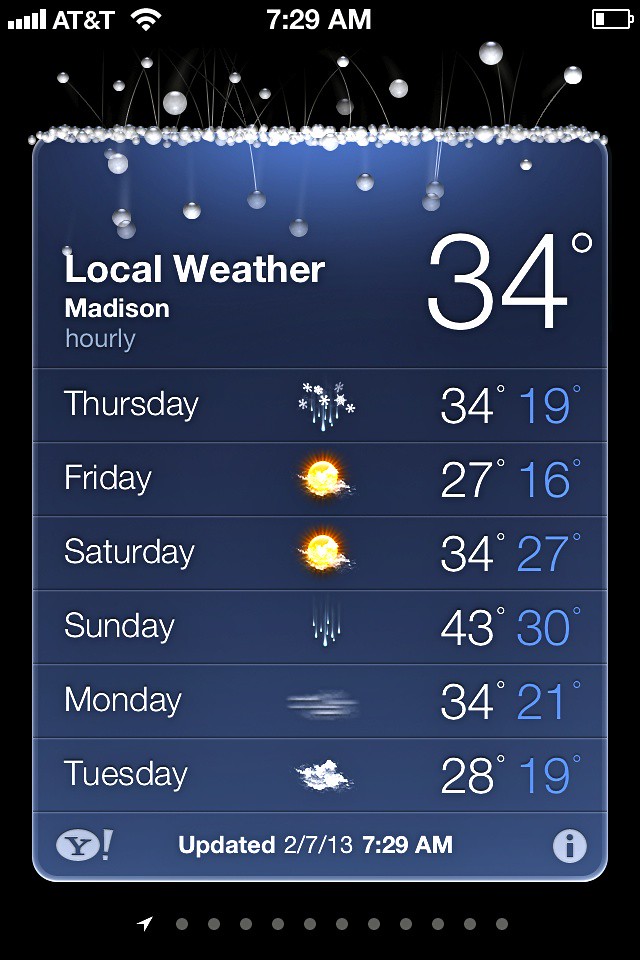This detailed screenshot from an AT&T phone shows a display of full bars for both cellular and Wi-Fi signal at 7:29 AM, with a battery level at approximately 25%. The local weather in Madison at the time is snowy with a temperature of 34 degrees. The weather information is displayed within a rectangular section topped with animated snowflakes and snowballs bouncing around but remaining in place. The forecast for the coming days is as follows:

- **Thursday**: Snowy, high of 34°F, low of 19°F.
- **Friday**: Mostly sunny, high of 27°F, low of 16°F.
- **Saturday**: Mostly sunny, high of 34°F, low of 27°F.
- **Sunday**: Rain showers, high of 43°F, low of 30°F.
- **Monday**: Windy, high of 34°F, low of 21°F.
- **Tuesday**: Cloudy, high of 28°F, low of 19°F.

Beneath the weather information, there is a Yahoo logo on the left indicating the source and time of the last update (7:29 AM). In the middle, "729 AM" is displayed, and on the right, an information icon is present. Below this section, the interface shows options to scroll through 11 different pictures, charts, or pages. This comprehensive view contrasts the local snowy weather with the detailed upcoming forecasts and associated icons.